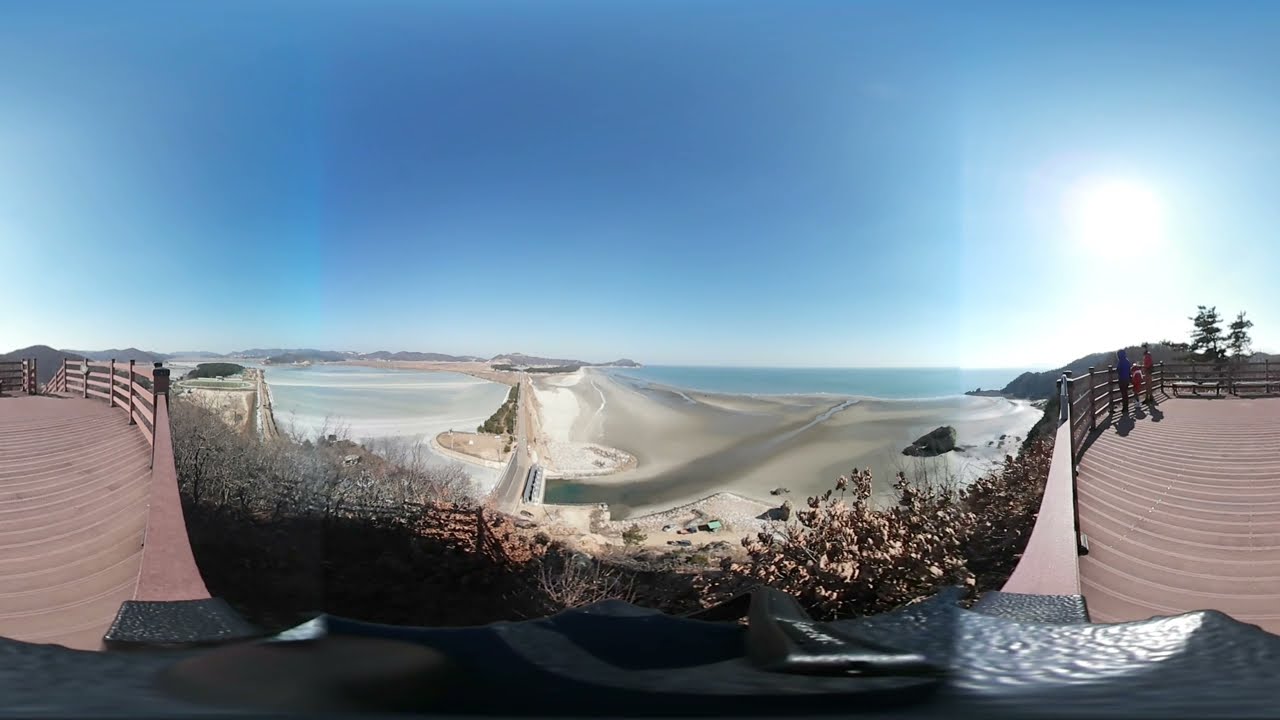This is a wide rectangular panorama photo of an ocean and beach taken from a high vantage point, possibly from a dock or wood walkway on a hill. The dock, appearing distorted due to the panoramic shot, stretches into the left and right corners of the image and consists of reddish-brown wooden slats with a fence running along its side. On the right side, three people stand against the fence, gazing out over the scene. 

In the foreground, a black, somewhat reflective surface is visible, featuring several dead plants. Below this viewpoint, you can see the beach's sandy banks and the expansive ocean. A river inlet and a dam are also visible at the bottom middle part of the picture. 

On the right side, beneath the bright, shining sun, there's another hill with green vegetation. The sky is a clear, cloudless blue. Far off in the distance, you can make out an island dotted with cottages or huts and some parked cars, enhancing the sense of depth and scale in the image.